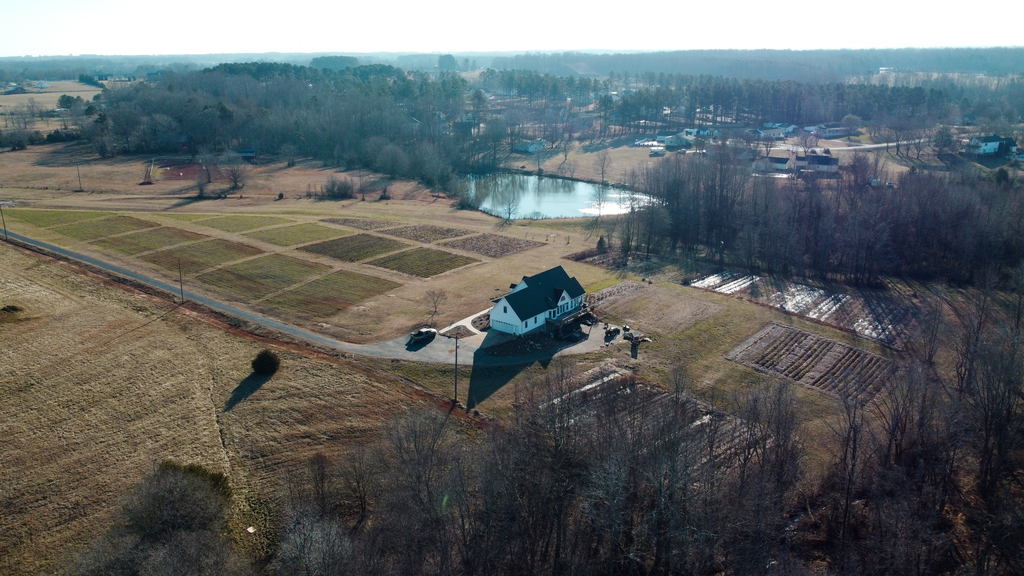The image presents an aerial view of an impressive white farmhouse with a black pitched roof, situated on expansive flat land. In the foreground, there's a connected garage section and a circular driveway with a car parked in it, leading to a narrow roadway on the left. The property occupies approximately one to two acres of land, divided into multiple sectioned-off portions possibly used for planting various crops. Eight distinct garden plots exhibit various colors—mostly greens and purples—indicative of different plant types. A small, triangular pond flanked by a grove of barren trees sits prominently to the right of the house, suggesting a winter or fall setting. Surrounding the farmhouse are more trees and some additional outbuildings. In the background, the landscape reveals a community of additional homes and farmhouses, providing a sense of the broader rural setting. The aerial perspective, likely captured by a drone or airplane, underscores the detailed layout and expansive nature of the farmland.